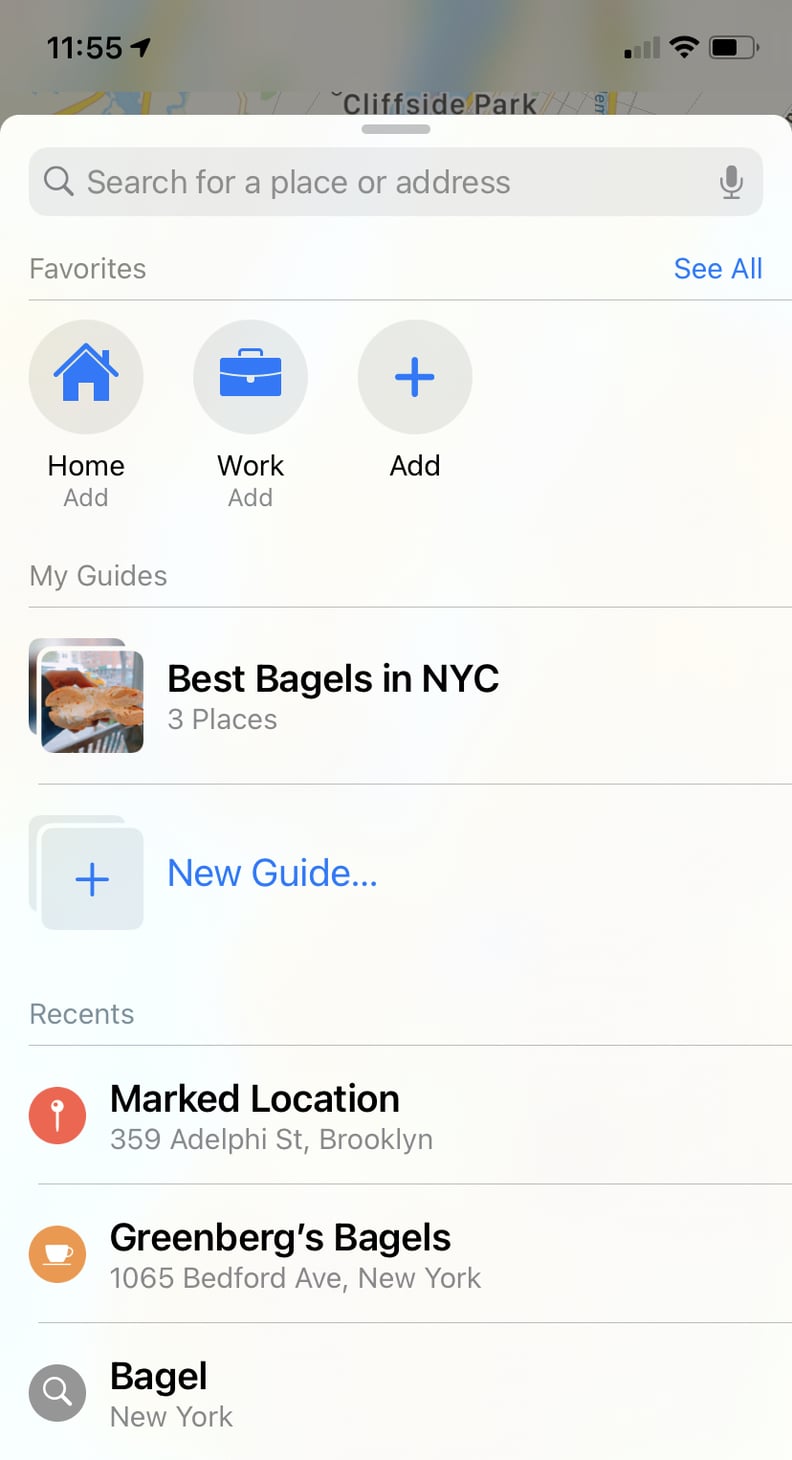In this screenshot from a smartphone's Maps app, the interface is meticulously detailed. At the top, a search bar prominently displays the text "Search for a place or address." To the right of this bar is a mic icon, while a search icon resides on the left side. Below the mic icon, a blue button labeled "See all" is clearly visible. 

A section titled "Favorite" follows, featuring three icons: a blue house representing "Home," a blue briefcase for "Work," and a blue plus sign for adding new locations. Just below these, a category named "My Guide" lists "Best Bagels in NYC," which includes three places. Another entry, "New Guide," is noted in black text accompanied by a blue plus sign. 

At the bottom of the screen, under the "Recent" section, there are three marked locations: "359 Adelphi Street, Brooklyn," indicated by a red icon with a white key; "Green Bags Bagels" at "1065 Bedford Avenue, New York," marked by an orange icon with a white cup; and "Budget New York," identified by a gray icon with a white search icon. Each icon serves as a visual reference to the associated location, enhancing the navigational experience within the app.